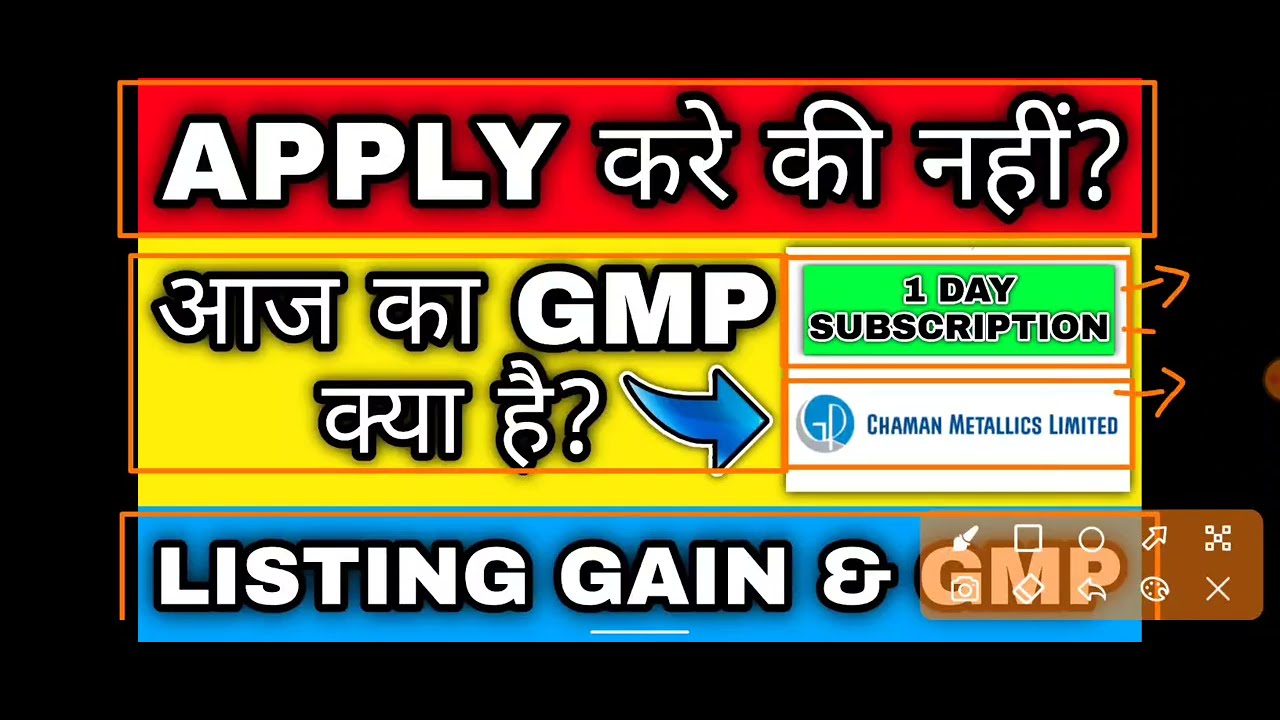The image appears to be an advertisement displayed on a computer screen, identifiable by a menu in the bottom-right corner suggesting options for editing or drawing on the image. The composition is structured around a central rectangular section divided into three colored bars, each containing text in various languages and styles.

At the top of the central section, over a red background, the word "Apply" is prominently displayed in white font alongside some Oriental characters. The middle section features a yellow background with more foreign characters and the letters "GMP." To the right of this section, there is a small green background area with the phrase "One Day Subscription" in black font. The bottom section has a blue background, presenting the text "Shaman Metallics Limited" and another smaller blue area stating "Listing Gain and GMP." 

Additionally, the entire central section is circled or highlighted with an orange border, with three arrows originating from the middle section and pointing to the right, further emphasising certain aspects of the advertisement.